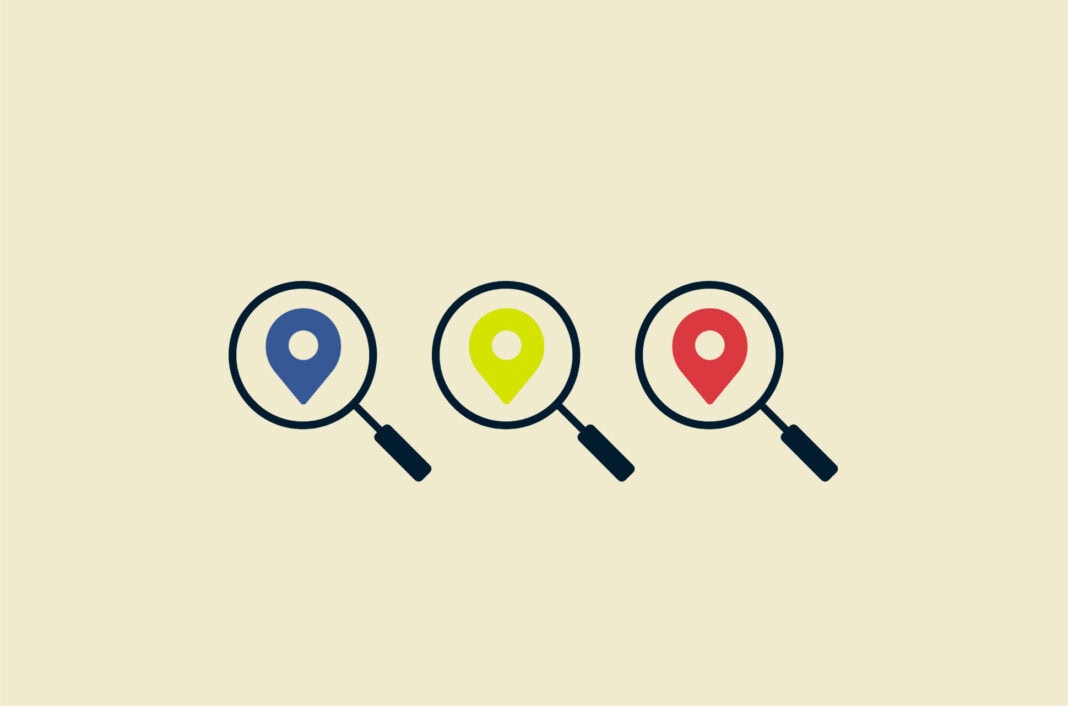This image is a detailed, computer-generated illustration set against a light beige backdrop. It features three identical black magnifying glasses, each positioned with their handles extending downward at a slant. The magnifying glass on the left encloses a blue teardrop-shaped design with a white circle inside. The middle magnifying glass contains a bright green or lime-colored teardrop design, also with a white circle. The magnifying glass on the right displays a red teardrop design with a similar white circle. These elements are centrally aligned in the image, and the overall composition is devoid of any text, emphasizing the stark, minimalist arrangement.